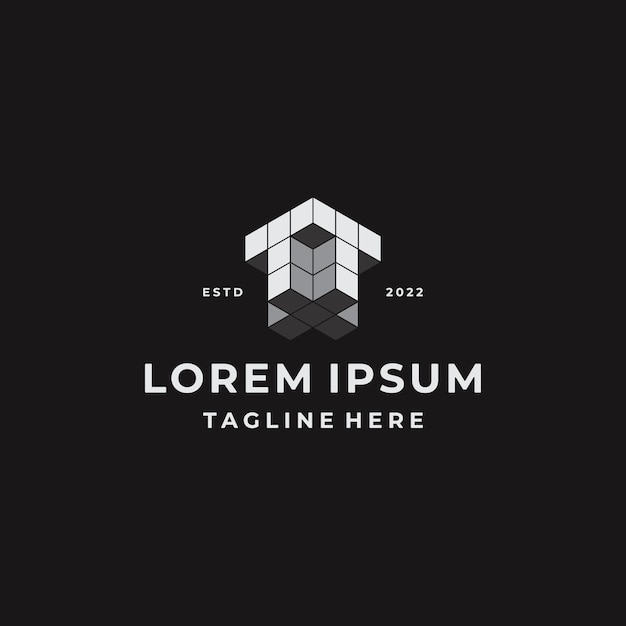This image showcases a 3D logo design on a jet black square background. The centerpiece is a meticulously shaded geometric composition of four three-dimensional letter T's, each constructed from five cubes—three cubes across and two cubes down—forming an intricate structure where the bottoms of the T's join into an X shape, and the tops create a square. The shading in white, gray, and black provides a dynamic depth, highlighting the top T's that face the viewer diagonally, revealing the bottom of this object. To the left of this central emblem, the letters "ESTD" appear in small white text, with "2022" mirrored on the right side. Beneath the logo, in larger white sans-serif font, is the placeholder text "Lorem Ipsum," followed by "tagline here" in slightly smaller sans-serif font. This overall composition suggests a template for a logo and tagline, commonly used in design presentations for its use of standard placeholder text and stark, modern aesthetic.